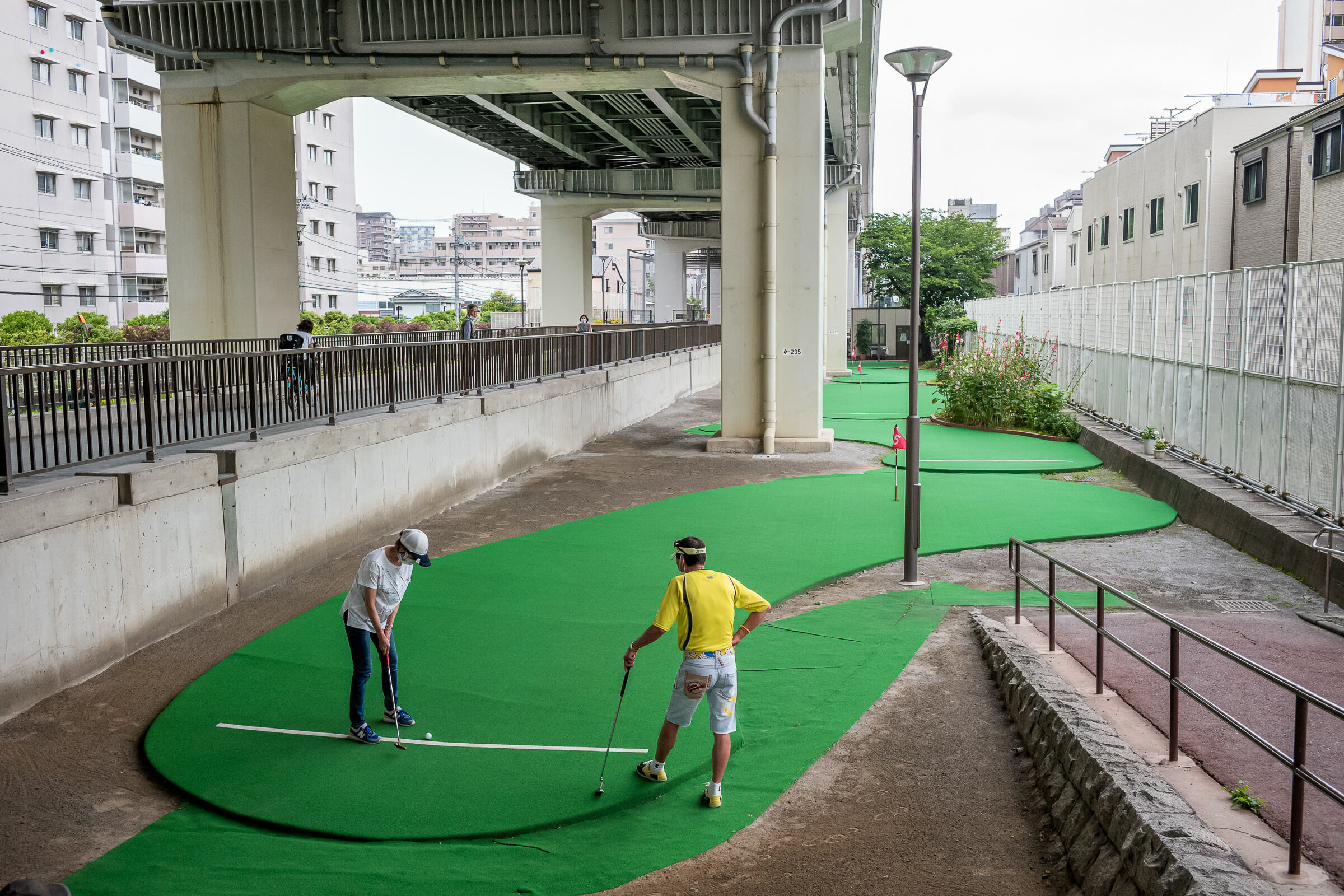In this image, we see two men playing golf on a unique, man-made course situated beneath a bridge. The golfer on the right, dressed in a yellow shirt, blue jean shorts, white socks, and sneakers, sports a headband and rests his right hand on his hip while holding the golf club with his left hand. The golfer on the left, wearing a white shirt, blue jeans, and sneakers, is poised to hit the ball, with a baseball cap adorning his head. The setting appears urban, with a sidewalk to the left featuring a person looking down on the golf players and another individual riding a bicycle behind them. The course, laid atop cement, is enclosed by a chain-link fence on the right, beyond which lies a building with a single window per section, and a tree at the far left. Also notable are three additional flags denoting separate holes on the course, a streetlamp amidst the greenery, and various railings and pathways, implying this could be a putt-putt course integrated into an urban environment, surrounded by buildings and elevated pathways.